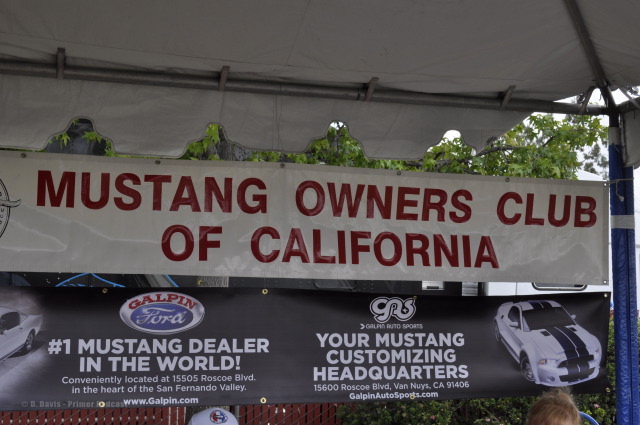This horizontally oriented photograph depicts a lively outdoor scene set under a large canvas-topped structure supported by steel railings. Dominating the space is a prominent sign that reads "Mustang Owners Club of California" in bold red text. Beneath this, a second sign declares "Galpin Ford, number one Mustang dealer in the world" and proudly states, "Your Mustang Customizing Headquarters," accompanied by additional details including an address and website. The banners are part of a setup typical for a Mustang Owners Club gathering, highlighting an image of a sleek white Mustang with a black racing stripe. The cheerful ambiance and bright summer day suggest a perfect occasion for car enthusiasts to convene and celebrate their shared passion. The detailed background of the sign is black, making the text and imagery stand out vividly against the crisp outdoor atmosphere.